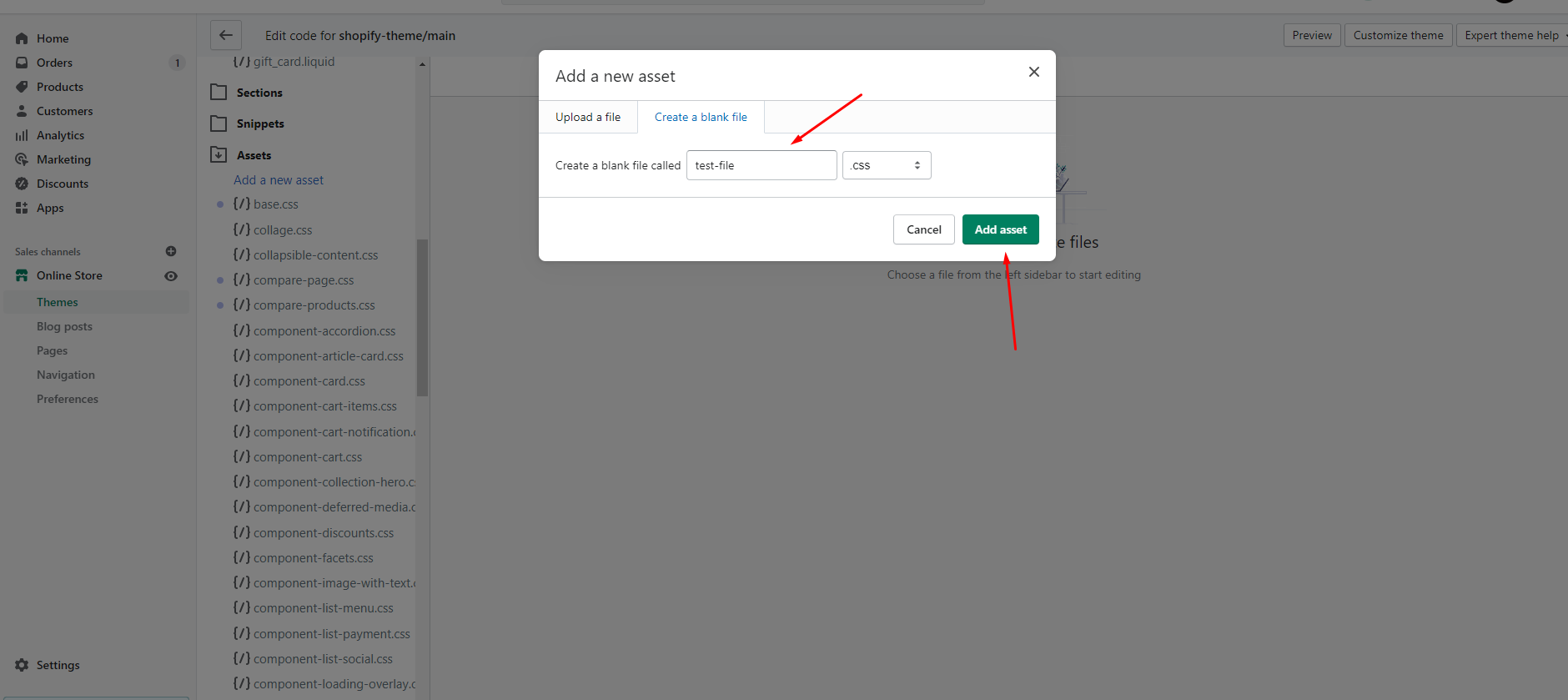This is a screenshot of what appears to be an online store interface, potentially a platform like Shopify, although the exact platform is not confirmed. The majority of the interface is grayed out, focusing attention on a white overlay panel. This overlay features multiple options: "Add a New Asset," "Upload a File," "Create a Blank File," and an indiscernible option with tiny text. A red arrow points towards the text, which mentions "CSS," suggesting a focus on style sheet management. At the bottom of the overlay, there are two buttons: a "Cancel" button on the left and a green "Add" button on the right.

Underneath the grayed-out interface, the left sidebar menu remains visible, listing navigational options: "Home," "Orders," "Products," "Customers," "Analytics," "Marketing," "Discounts," and "Apps." Below these, separated by a break, are additional options under "Online Store" including "Themes," "Blog Pages," "Pages," "Navigation," and "Preferences." To the right of the sidebar, there's a column displaying a file system, which includes directories like "Snippets" and "Assets." The assets seem to be primarily CSS files, though the text is too small to read clearly.